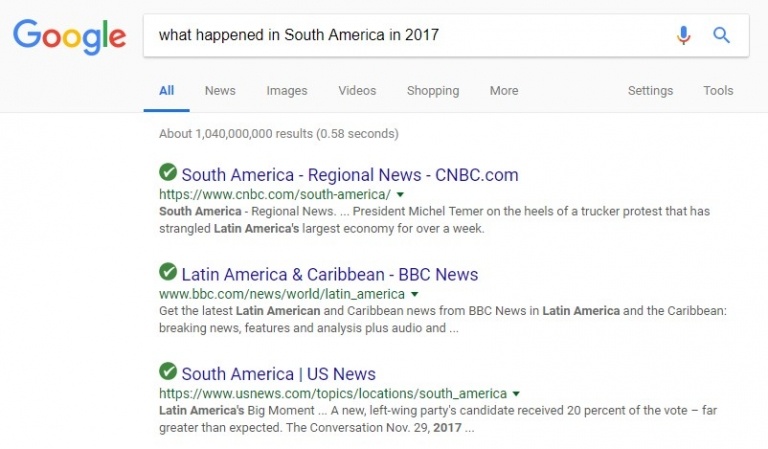The image depicts the Google search home page, prominently featuring the word "Google" spelled out with each letter in its distinct color: the first "G" in blue, the first "O" in red, the second "O" in yellow, the small "g" in blue, the "L" in green, and the "E" in red. Positioned centrally beneath the logo, the search bar displays the query "what happened in South America in 2017," highlighted in blue with a blue underline.

Below the search bar, navigation options—News, Images, Videos, Shopping, More, Settings, and Tools—are displayed in gray text. Further down, the search results begin, showing approximately 1,040,000 results in 0.58 seconds.

The first highlighted result, credited to CNBC, includes a green check mark and mentions a significant event involving President Michael Turner amid a trucker protest disrupting Latin America's largest economy for over a week. The associated website is www.cnbc.com/SouthAmerica.

The second highlighted result from BBC News, also marked with a green check, focuses on Latin America and the Caribbean. It promises comprehensive coverage, including breaking news, features, analysis, and audio content, with the URL www.bbc.com/news/world/latin_america.

The third highlighted result from US News, again ticked with a green check mark, discusses a political development in Latin America where a new left-wing party candidate unexpectedly garnered 20% of the vote. The relevant link is www.usnews.com/topics/locations/SouthAmerica.

The backdrop of the page is predominantly white, with the text presented in a purplish-gray hue.